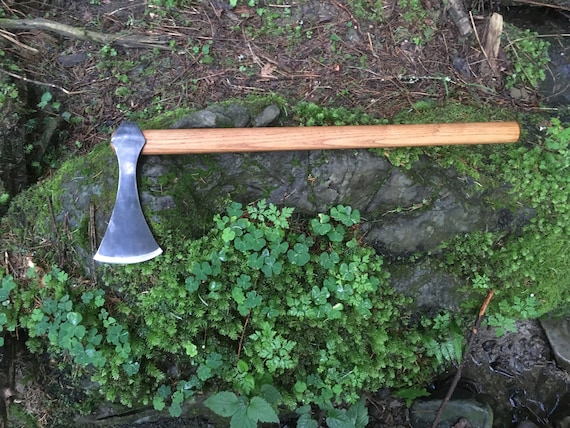The outdoor image, taken from an overhead perspective, features a hand axe resting atop a large, moss-covered boulder embedded in dark gray soil. The axe, with a finely finished, light brown wooden handle, has a small, narrow-headed, silver metallic blade that curves outward at the edge. Surrounding the boulder and axe are patches of green clover and sporadic foliage, including some small green vines and sticks scattered across the ground. The edges of the photo have a darker tone, accentuating the natural setting of dirt and rocks. Despite its formidable appearance, with the blade beveled and designed to cut, the axe seems more decorative, reminiscent of a medieval war axe.